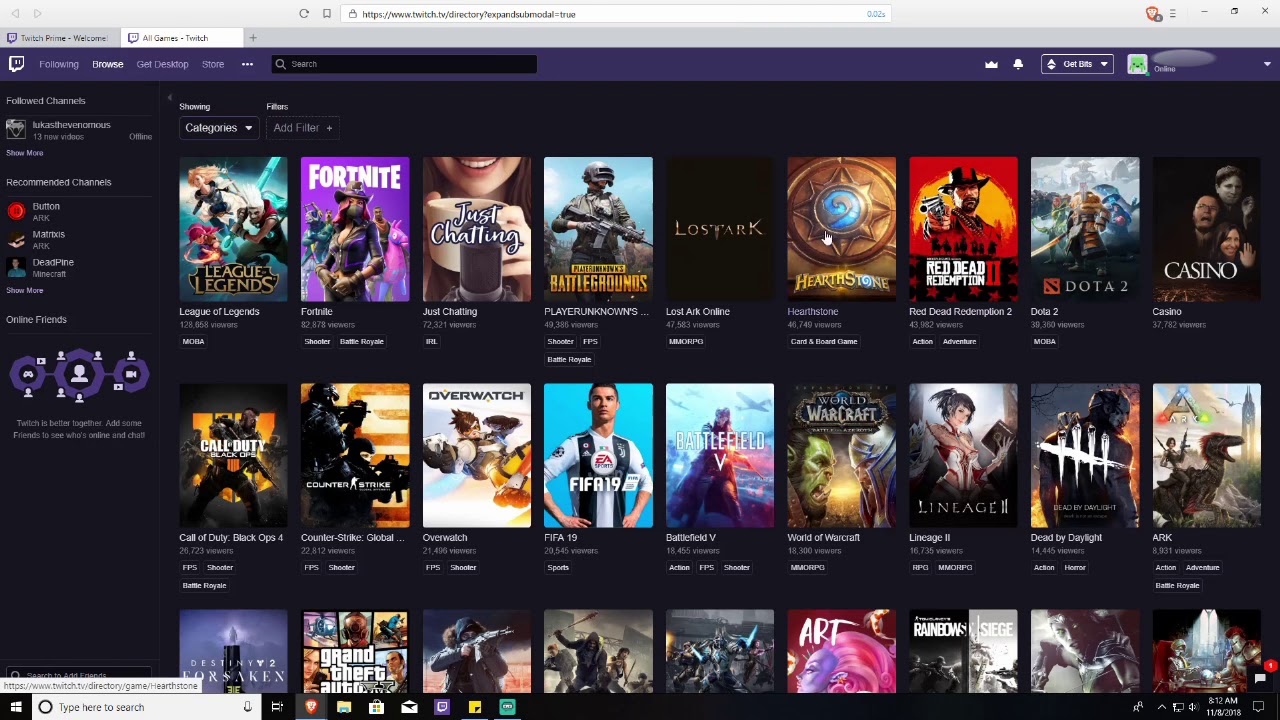The image depicts a computer screen displaying a website featuring a selection of games. The browser interface shows two open tabs, with the active tab being the second one. At the top of the screen, the URL is visible in a white search bar. Below, the main content area features a purplish-colored background with a black search bar. On the left-hand side, five categories are listed in white text against a dark gray backdrop. 

The left side of the screen also includes small, vertically-oriented text and three purple circles containing profile picture icons. 

The central and right portions of the screen display three horizontal rows of game thumbnails, each row showcasing nine games. The bottom row only partially reveals the game cover art, while the top two rows fully display the cover art along with the game titles in white text beneath each.

In the top right corner, there are several icons: a notification bell, a crown, an additional tab, a white square with green elements, and a gray oval. The bottom right corner displays computer system icons, including the current time.